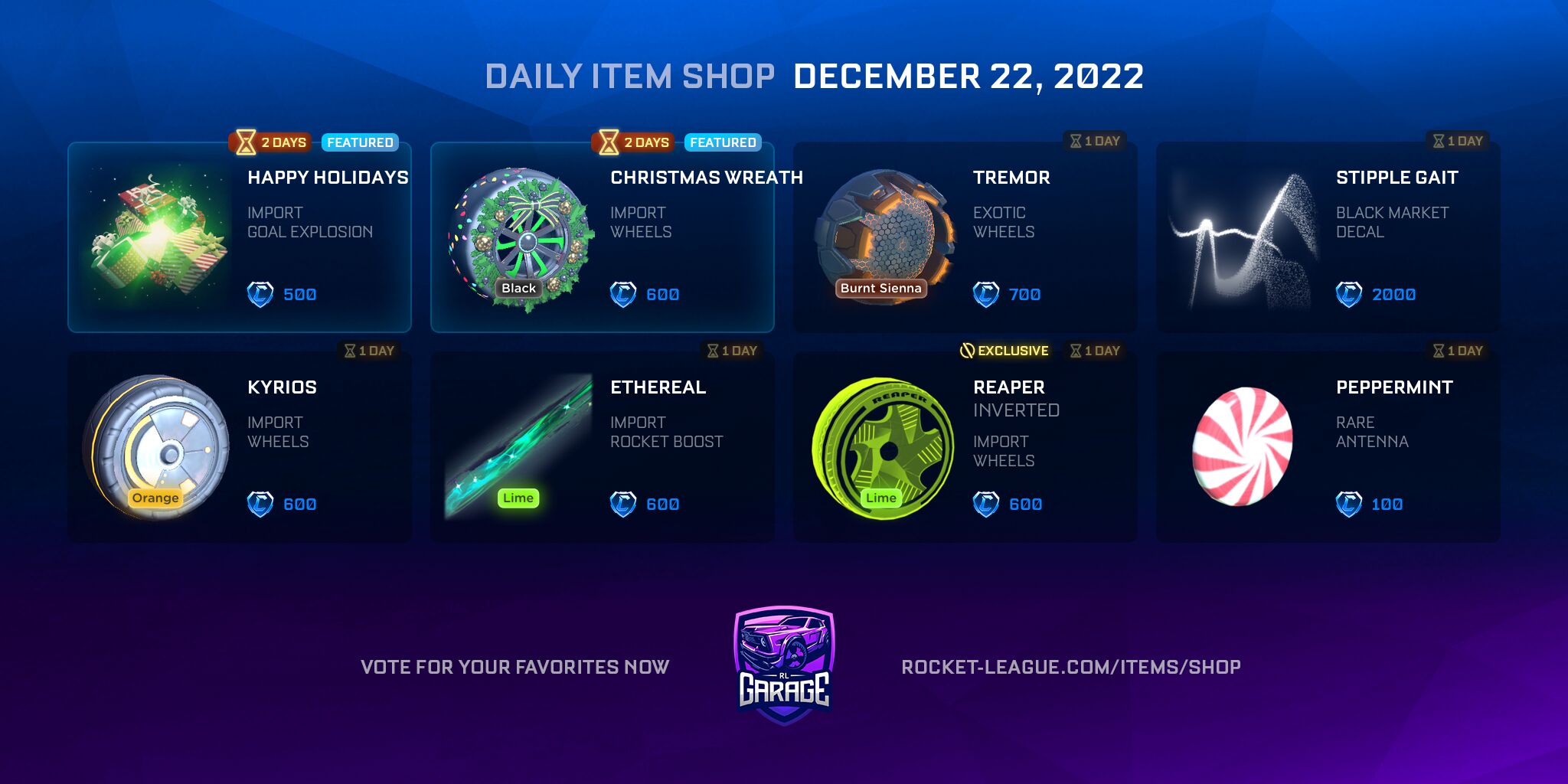Here is a cleaned-up and detailed caption for the screenshot of the Rocket League in-game menu:

---

Screenshot of the Rocket League Daily Item Shop for December 22nd, 2022. The menu showcases eight purchasable in-game items against a blue-to-purple gradient background. At the bottom of the image, there is a badge featuring a car and labeled "Garage," accompanied by the text: "Vote for your favorites now, rocketleague.com/item/shop."

The shop offers various cosmetic items for the cars used in the game, where players engage in soccer matches using rocket-powered vehicles. Available items include:

- **Christmas Wreath Wheel**: A festive wheel adorned with a Christmas wreath, priced at 600 of the in-game blue currency.
- **Exotic Wheel "Tremor"**: A unique and visually striking wheel available for purchase.
- **Peppermint Reaper Wheel**: A green and holiday-inspired wheel design.
- **Various Boost Effects**: Including ethereal effects to enhance car aesthetics.
- **Assorted Decals**: Customizable decals for car appearances.

Each item listing shows its price and the duration it remains available for purchase.

---